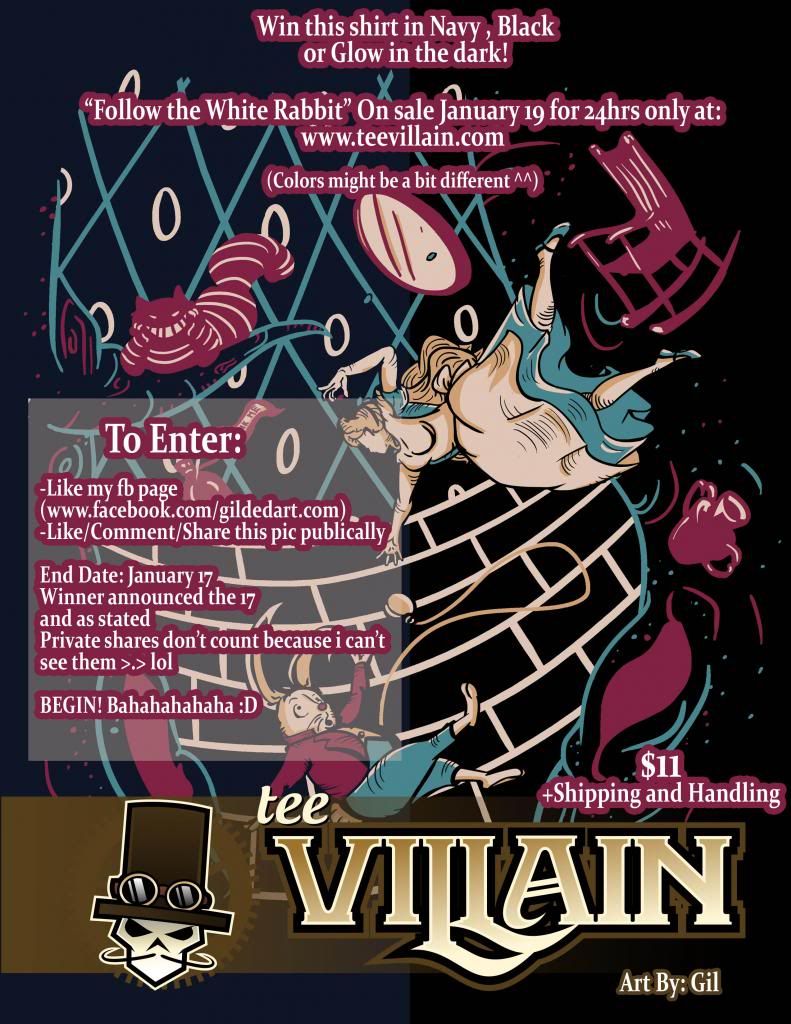**Descriptive Caption:**

This image resembles a vertical rectangular poster set against a background that transitions from a lighter black or even blue on the left side to solid black on the right. The main text area features white lettering embedded in a dark reddish backdrop, shaped to contour each letter. The prominent text reads: “WIN THIS SHIRT IN NAVY, BLACK, OR GLOW IN THE DARK!”

Below this text, another line, set apart by a small space, states: “Follow the white rabbit.” Further down, it mentions: “On sale January 19th for 24 hours only at: www.ttevillain.com (colors might be a bit different).”

The visual design contains intricate turquoise diamonds connected by off-white to yellowish ovals, within which lies a red-striped cat lounging with its chin resting on its paws. On the far right edge sits a deep red rocking chair. Adjacent to it, a tilted looking glass with a cream-colored mirror leans toward the bottom left corner. Alice from Alice in Wonderland, depicted in her signature blue dress, white apron, blue shoes, and sporting blonde hair, is illustrated falling sideways. Her feet point towards the upper right, her body aligns with the middle, and her hand reaches down gracefully.

On the lighter colored square on the left side of the image, white lettering over a red background reads: “TO ENTER: LIKE MY FB PAGE (www.facebook.com/gildedart). LIKE/COMMENT/SHARE THIS PIC PUBLICLY. END DATE: JANUARY 17TH. WINNER ANNOUNCED THE 17TH. PRIVATE SHARES DON'T COUNT BECAUSE I CAN'T SEE THEM. GREAT SIZE LOL. BEGIN! BAH: THREE DAY.”

Towards the bottom of the poster, there is a figure sporting a red long-sleeve top and blue pants, with bare feet, reaching up toward Alice. On the lower right corner, “$11 plus shipping and handling” is written. At the very bottom, the text “in ivory tee” is followed by “villain” in cream and slightly brown font with black borders. Finally, it is noted that the art is by “Gill,” next to a figure in a brown top hat with a long mustache.